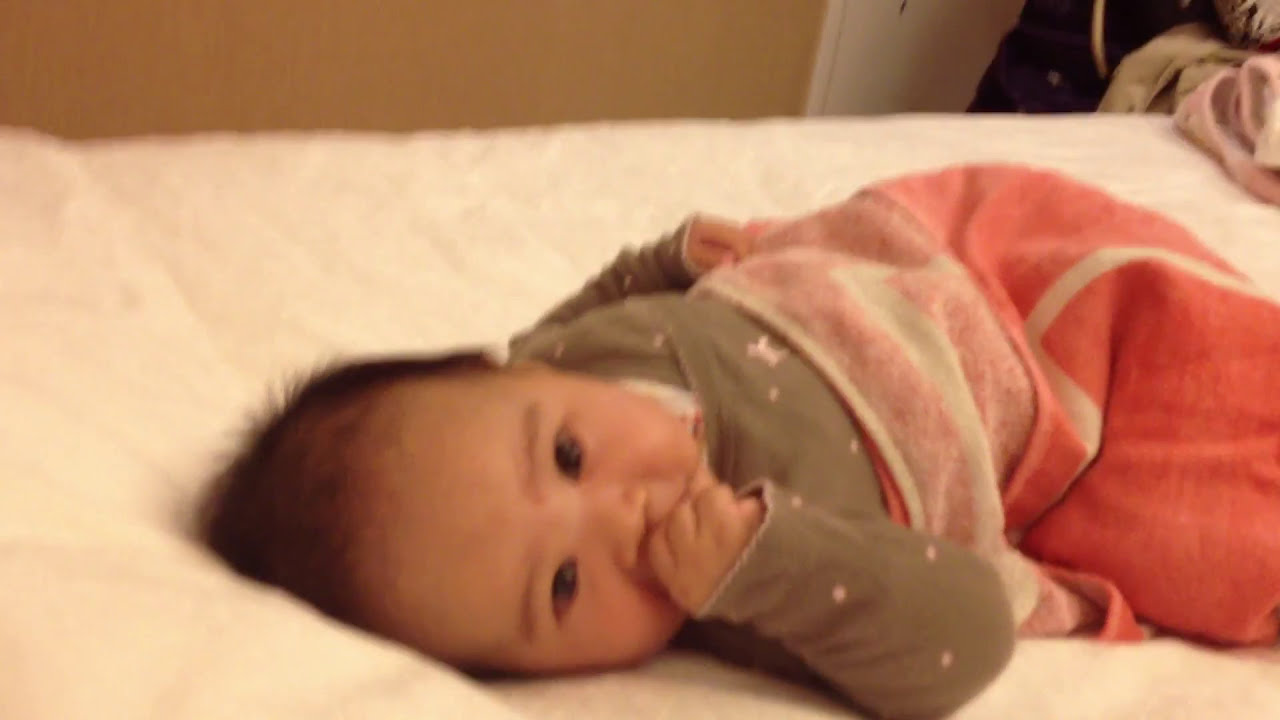In this detailed photo, an adorable Asian baby, approximately 6 to 8 months old, is lying on their back in a cozy bedroom setting. The baby has soft, wispy brown hair and is wearing a green shirt adorned with yellow markings, polka dots, and characters. Their chubby fist is raised to their mouth as if they might be sucking their thumb, a gesture that suggests contentment. Wrapped from the waist down in an orange and white striped blanket, the baby rests on a white bed, which is set against a beige wall. In the background, to the far right, there is a towel, and what might be a door, along with a few other items that could potentially be slippers or laundry. The baby's round face, big eyes, and puffy cheeks add to the endearing scene, evoking a sense of peacefulness and warmth.